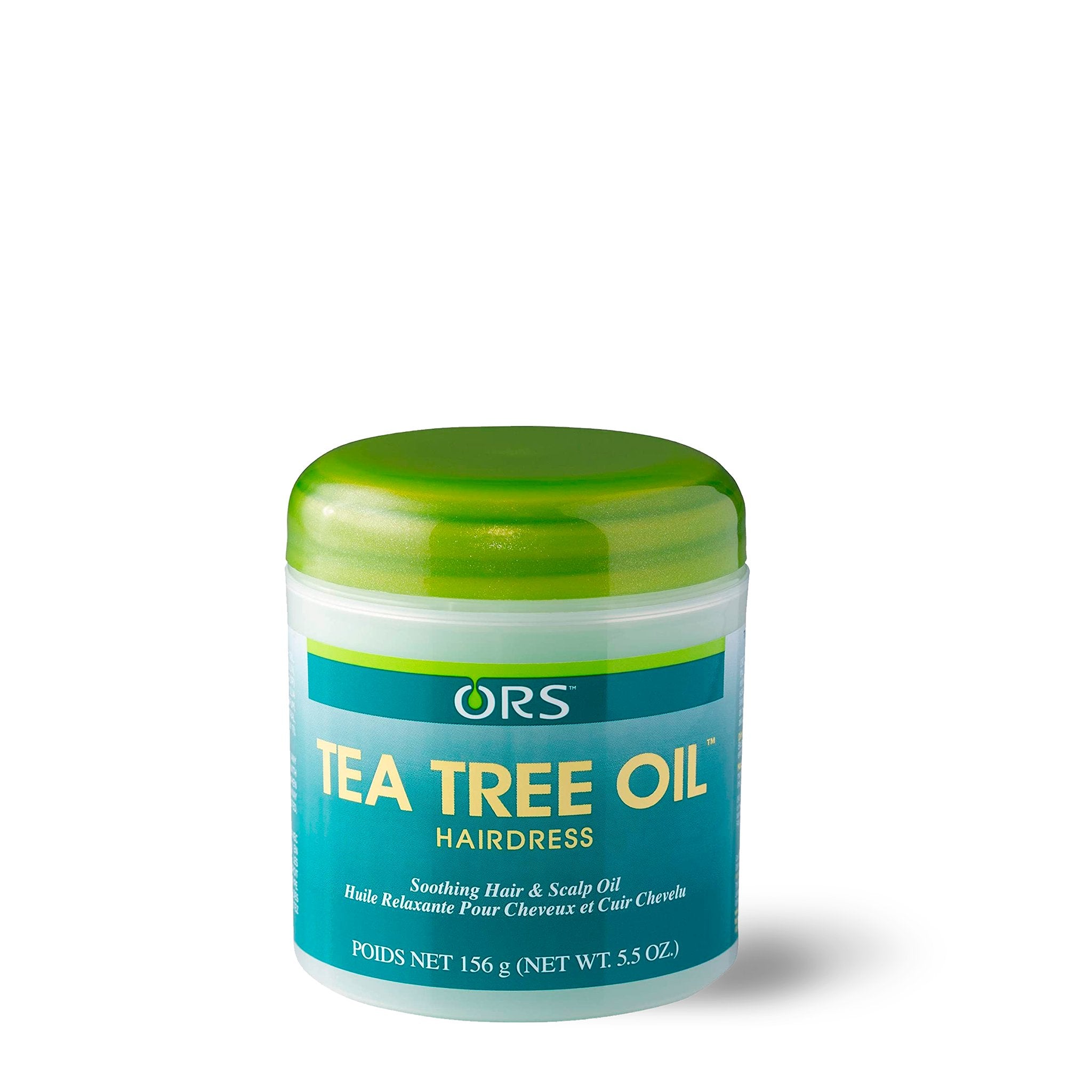The image features a close-up of a small, clear plastic container of tea tree oil against a white background. The container has a light green twist-off cap. The label is predominantly a gradient of blue and turquoise, becoming lighter towards the top. At the very top of the label, there is a green and turquoise rectangle with the letters "ORS" in white, incorporating a green teardrop shape inside the "O" that connects to a green horizontal band. Below this, in orange letters, it reads "Tea Tree Oil," followed by "Hairdress" in yellow. Further down, in white letters, it states "Soothing Hair and Scalp Oil," with the same text repeated in French underneath. At the very bottom of the label, it specifies "Net 156 grams, Net weight 5.5 ounces." The plastic container itself is clear, showcasing the contents inside.